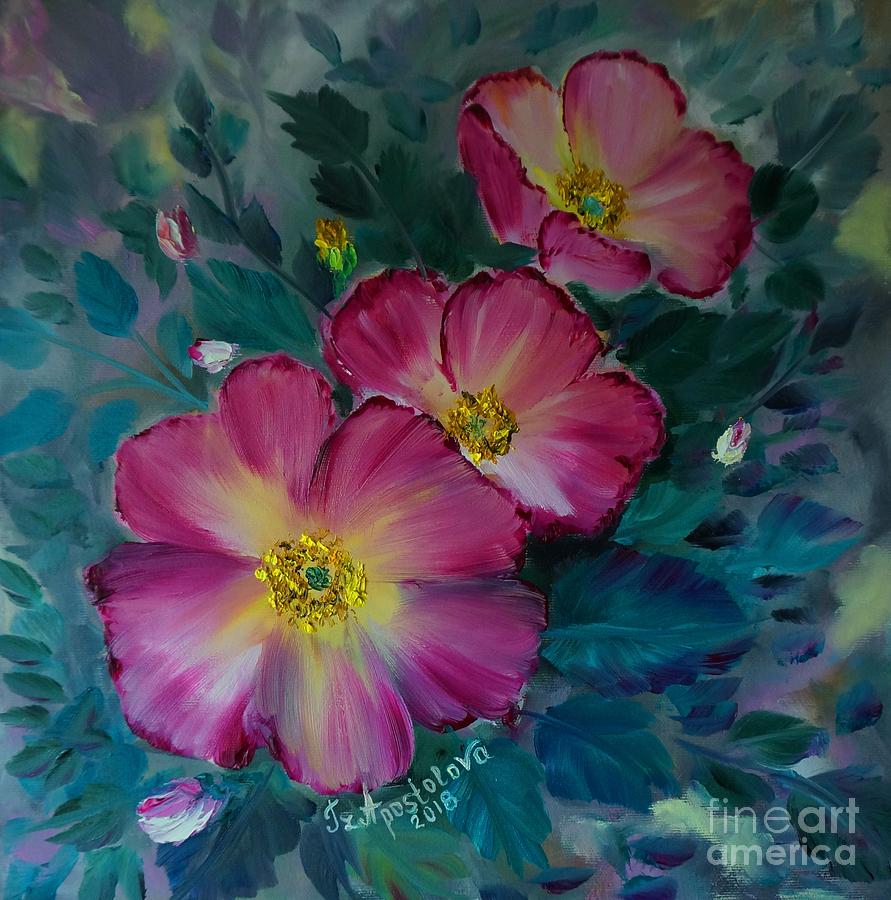This detailed oil painting features a striking composition of three vibrant pink flowers with yellow centers, radiating out to green at the very heart. The petals exhibit a beautiful gradient, transitioning from deep pink at the edges to a rich yellow at the core. The flowers are arranged diagonally, starting from the bottom left and extending to the upper right, against a lush backdrop of bluish-green leaves detailed with delicate vines. The closest flower at the left is fully visible, showcasing its intricate stamen and pistil, while the flower to its right is partially obscured, and the third flower, positioned at an angle, reveals both its back and front petals. This captivating piece also features a faint but bold "Fine Art America" logo in the bottom right corner, and is signed by the artist, Jet Paselova, with the year "2018" noted below the signature.